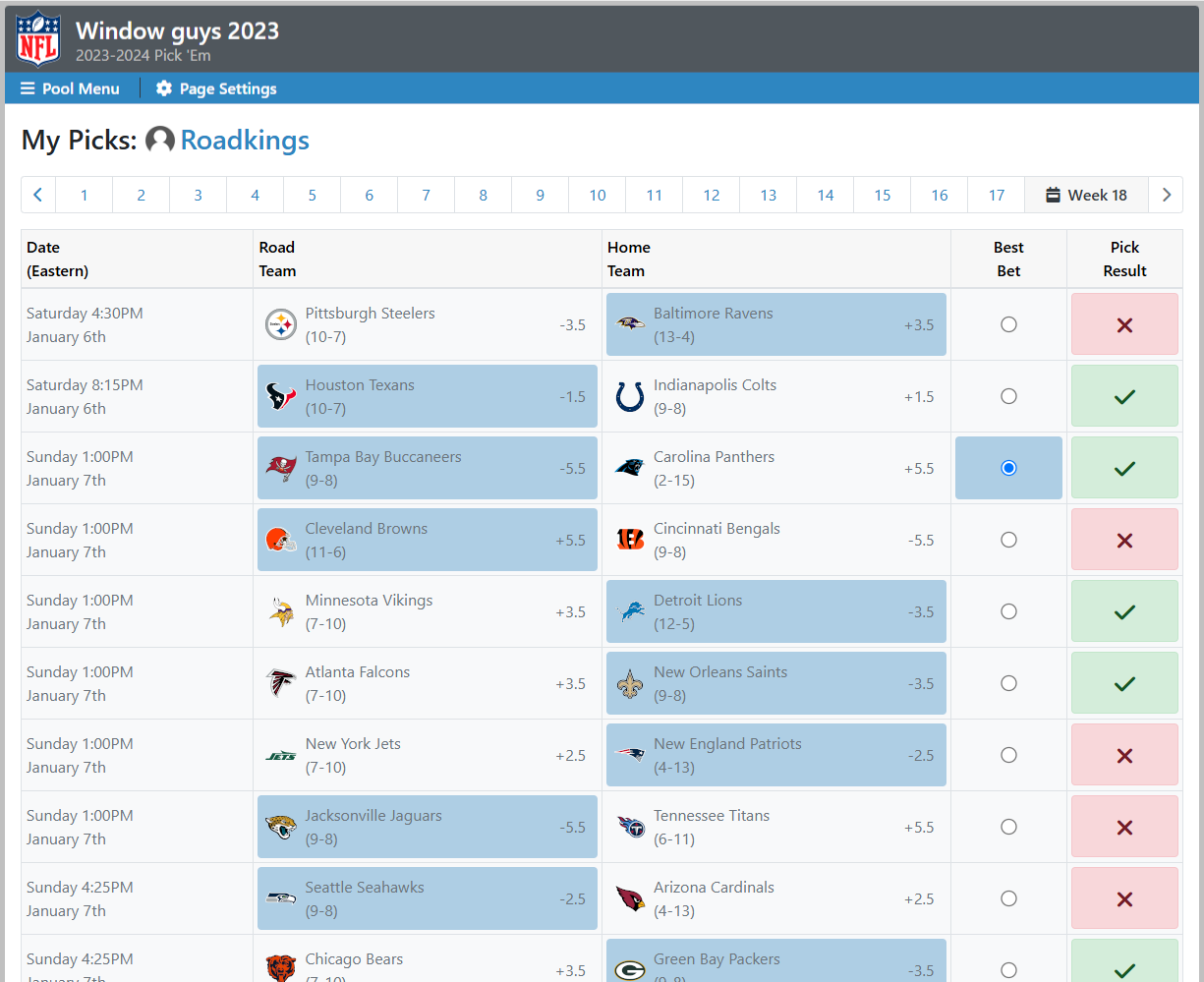The image displays a detailed schedule featuring NFL game picks with Josh Allen's mustache as an added thematic element. In the upper left corner, "My Pics: Josh Allen's - Mustache" is written in black text. Below that, the word "Date" is shown in parentheses, indicating Eastern Time, followed by specific game times: Saturday at 4:30 p.m., Saturday at 8:15 p.m., and three instances of Sunday at 1:00 p.m., extending down to Sunday at 4:25 p.m.

The next category is "Road Team," listing the Green Bay Packers, Pittsburgh Steelers, and Washington Football Team in blue rectangles. To the right, the "Home Team" column also lists teams in blue rectangles: Denver Broncos, Philadelphia Eagles, Minnesota Vikings, Cleveland Browns, Jacksonville Jaguars, Houston Texans, and Tampa Bay Buccaneers.

The final column, titled "Pick Result," indicates the outcomes with green checks and red X's. There is one green check, followed by a red X, then two more green checks, another red X, and five more green checks at the bottom.

Overall, the image meticulously lays out a schedule with teams and game picks, visually coded with checks and X's to represent results.